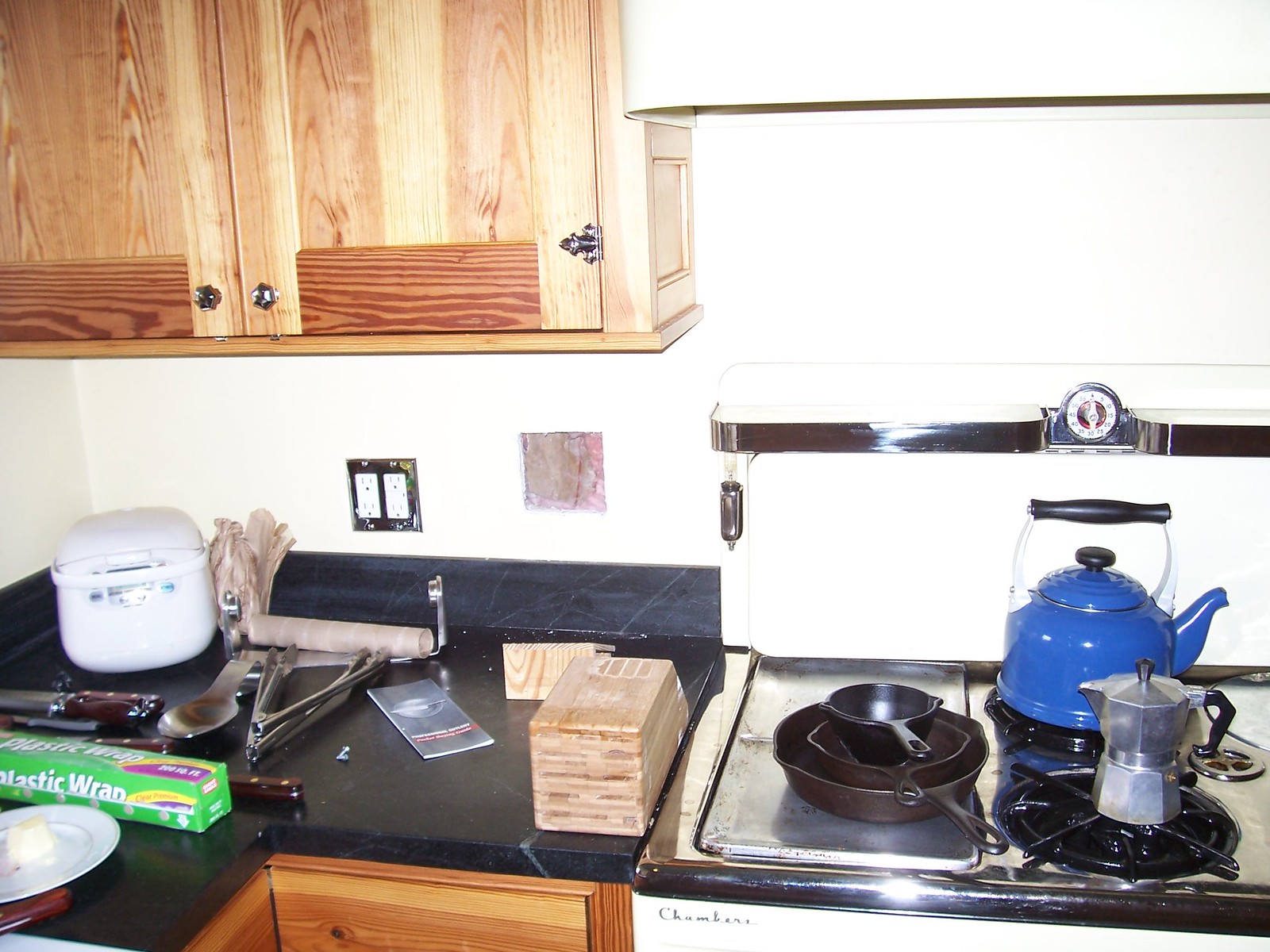The image portrays a kitchen scene with a focus on the stove and adjacent counter space. On the right side, there's a stovetop, presumably part of an oven unit not fully visible in the frame. The stovetop boasts a silver pan with two cast-iron skillets and a matching bowl stacked on top. A blue tea kettle rests on the back burner, and a coffee maker occupies the front burner, contrasting against the silver stovetop embedded in a white oven structure.

To the left of the stove, the countertop stretches out, forming a corner area. Here, a collection of kitchen items is scattered about: a rice cooker tucked into the far corner, a roll of saran wrap, a plate, two salad tongs, and a paper towel roll, which is unusually placed on the counter instead of mounted beneath a cabinet. Additionally, a pamphlet and a knife box, seemingly pushed over, add to the eclectic mix.

Above this corner space, there's a light brown pine wood cabinet fitted with silver hardware, appearing as a two-door unit. The scene captures everyday kitchen clutter, providing a glimpse into a casually organized yet functional cooking space.